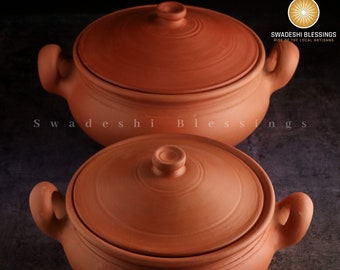This studio photograph captures two beautifully crafted terracotta clay pots, both adorned with matching lids equipped with small circular handles for easy removal. These pots, showcased against a dark backdrop, exhibit an earthy orange and brown color typical of terracotta, with chubby handles on both sides. The lids feature distinctive rivets, telling of their creation on a pottery wheel. The pot in the foreground is slightly less visible, while the one in the background, closer to the center, reveals its full, wide, and stout form. A prominent logo in the corner showcases a yellow sunburst with white rays and the text "Swadeshi Blessings" in bold, white block letters. Additionally, the image has semi-transparent text with wide spacing across the center, also stating "Swadeshi Blessings." This photograph, possibly designed for advertising, emphasizes the craftsmanship and traditional beauty of these clay pots, making it a perfect candidate for featuring in a magazine or promotional material.